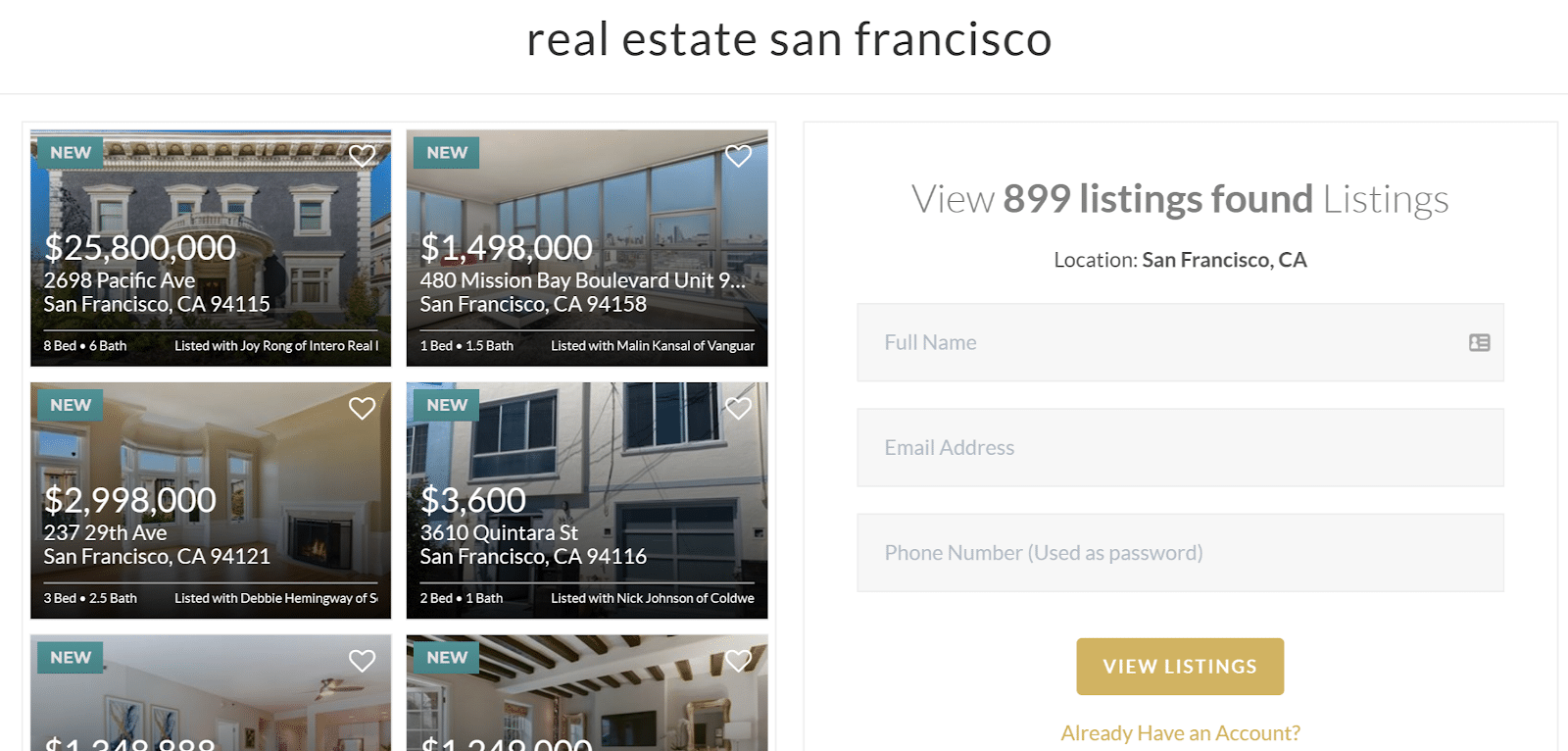The top portion of the image features a white background with the text "Real Estate San Francisco" in black, though "San Francisco" is not capitalized as one might expect. Below this, a thin gray line runs horizontally across the image. On the right side, there is a gray rectangle truncated at the bottom, making its full length indeterminate. Within this rectangle, bold text in gray states "View 899 listings found." Below this, in regular text with a capitalized 'L,' the word "Listings" is written.

Further down, in gray rectangles, there are three labeled fields: 
1. "Full Name," with each word capitalized.
2. "Email Address," with both 'E' and 'A' capitalized.
3. "Phone Number (used as password)," with initial capitals for 'Phone' and 'Number.'

Beneath these fields, there is a brownish-gold rectangle with white text that says "View Listings." Below this button, the text "Already have an account?" appears.

On the left side of the image, six property listings are presented. Each property has a tag in the upper left corner indicating "New" in white text. The properties listed show various prices:
1. $25,800,000
2. $2,998,000
3. $3,000,000 (partially cut off, showing only "3,000")
4. $1,498,000